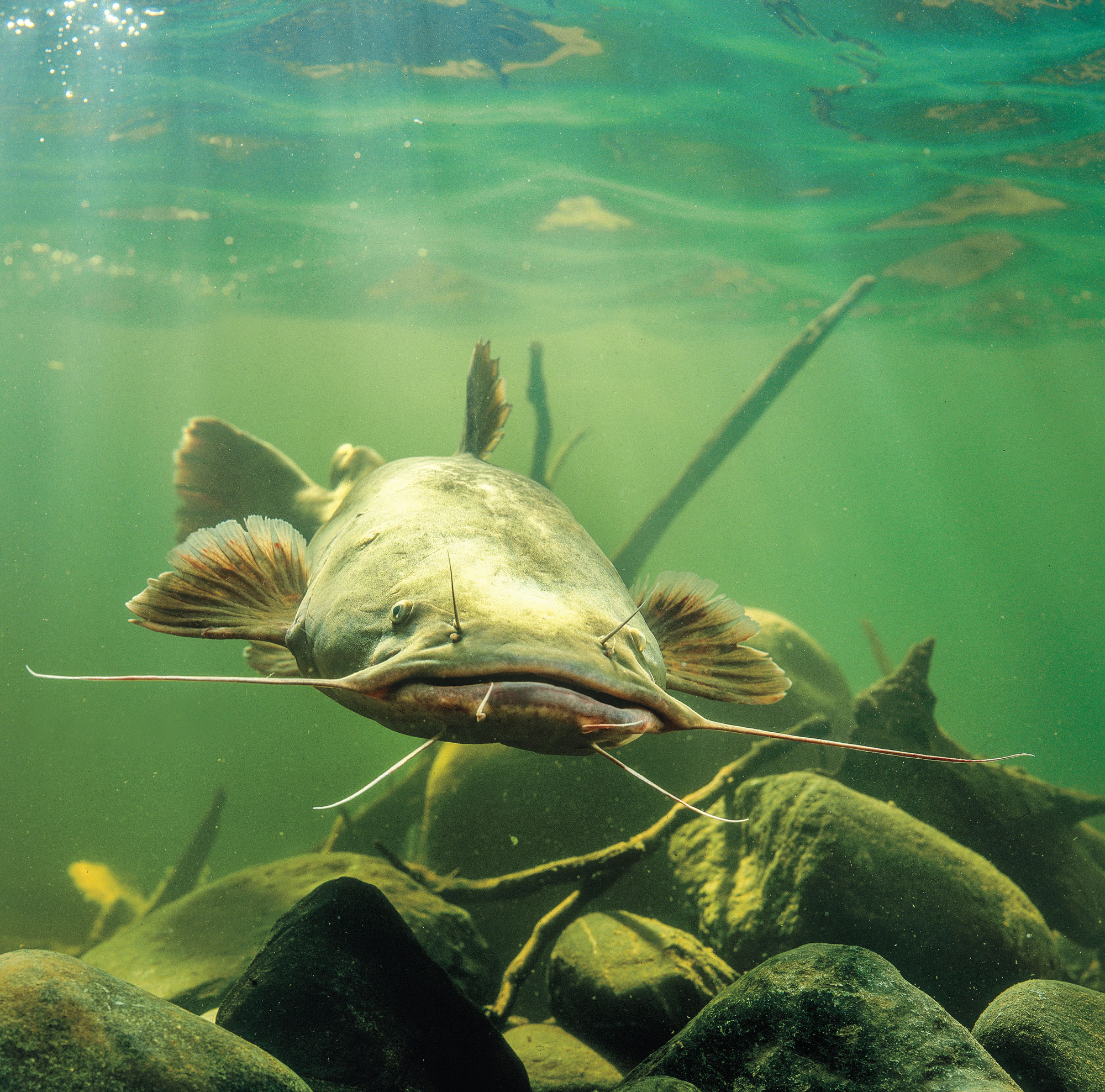This underwater photograph captures a detailed scene featuring a large hammerhead shark, gracefully swimming just above a bed of fairly good-sized rocks. The setting is suffused with a green hue, likely influenced by the environment, making the surrounding water and rocks appear green as well. The shark, distinguished by its iconic flat head with wing-like extensions on either side of its mouth, also looks green under this light. It features two small fins just behind its eyes, two more further back, and a distinctive dorsal fin situated towards its rear. Long, spiny whiskers are prominently visible around its mouth, chin, and by its nostrils, adding to its impressive appearance. In addition to the rocks, the bottom of the riverbed or aquarium showcases a piece of wood extending well into the water and a stick resting among the stones. Sunlight filters down from the water's surface, illuminating the back of the shark and highlighting its motion. Overall, elements like the shark’s movement, the sunlit water, and the detailed backdrop of rocks and wood create a vivid and dynamic underwater scene.